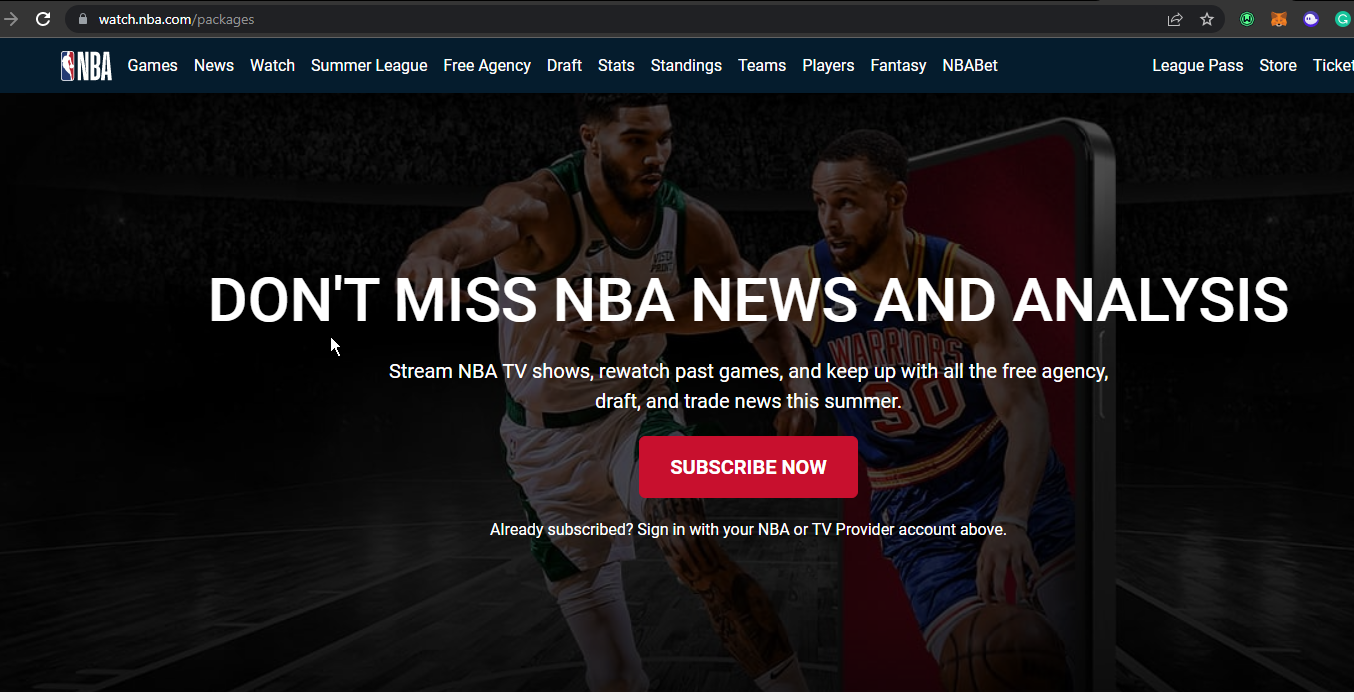The provided image shows the homepage of the website watchNBA.com/packages. At the top of the page, there is a navigation menu with the iconic NBA logo located on the far left. The menu, designed with white text on a navy blue background, features several links to different sections of the site. These links, from left to right, are labeled: Games, News, Watch, Summer League, Free Agency, Draft, Stats, Standings, Teams, Players, Fantasy, NBA Bet. Further to the right are additional links for League Pass, Store, and Tickets.

Dominating the center of the webpage is a large red button with white text that reads "Subscribe Now." This button is prominently placed to attract user attention. The background behind the button is slightly darkened, depicting an intense moment in an NBA game. In this background image, two professional NBA players are in action. One of the athletes, dressed in a white uniform with green trim, is facing off against another player who is wearing a blue uniform with yellow accents. The latter player’s uniform clearly displays the team name "Warriors" and the number "30," indicating the player is a member of the Golden State Warriors, specifically Stephen Curry.